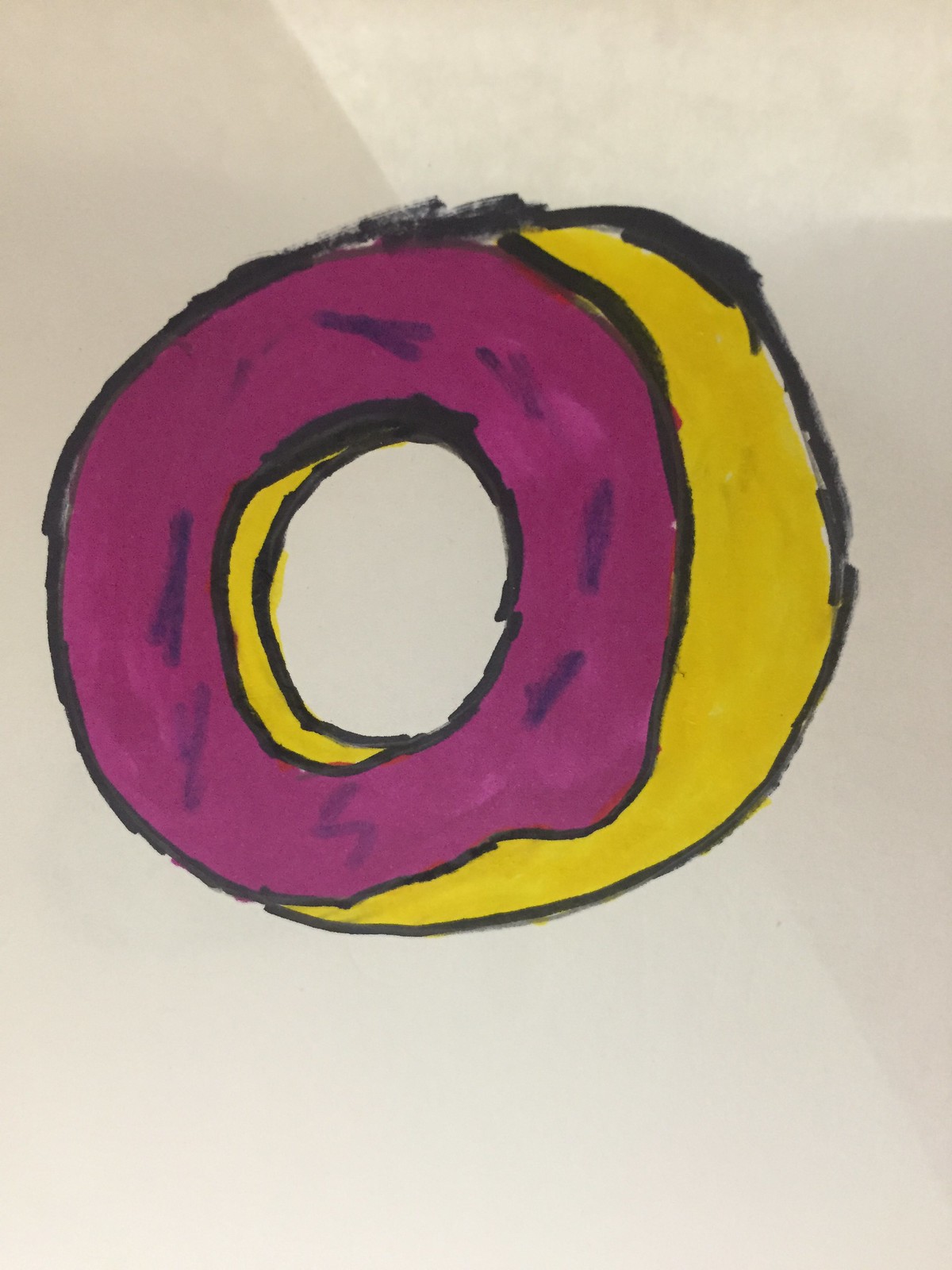The image is a vertically aligned portrait-style photograph of a roughly sketched donut on white paper. The donut is depicted in a three-dimensional, circular shape, drawn with a black marker outline. The front part of the donut is colored in shades of pink, purple, and maroon, with some darker lines scattered across the surface. The back and inside of the donut are filled with yellow. The drawing has a crude, childlike quality and appears hastily colored, possibly with felt-tip markers, giving it an unfinished look. The donut is shown from a side profile, facing towards the left, emphasizing its 3D appearance.